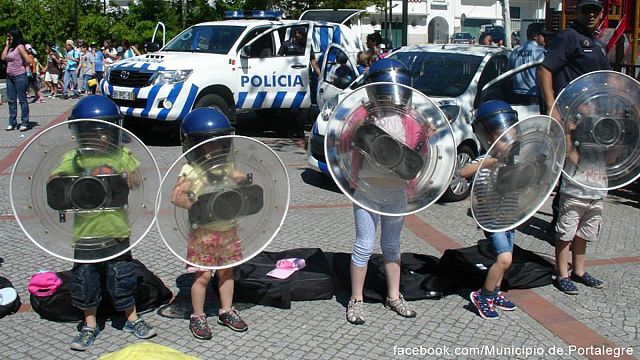The photograph captures a vibrant scene featuring five children, estimated to be between the ages of 4 and 8, standing in a row from left to right. Each child is equipped with child-sized blue police helmets that include clear face shields, and they are holding large, circular clear shields with black rectangular holders in the center, which likely have two handles. Dressed in their normal clothes but adorned with these police safety gear pieces, the children stand confidently in front of two white police cars adorned with blue stripes and the word "POLICIA" on the sides. Both vehicles have their front doors open, and their blue and white lights are visible on the roof. Black bags are neatly placed by the children's feet. In the background, several police officers are present near the cars, and a crowd of people can be seen mingling. The bottom right corner of the image features text that reads "Facebook.com/Municipio.de.PortoAlegre."